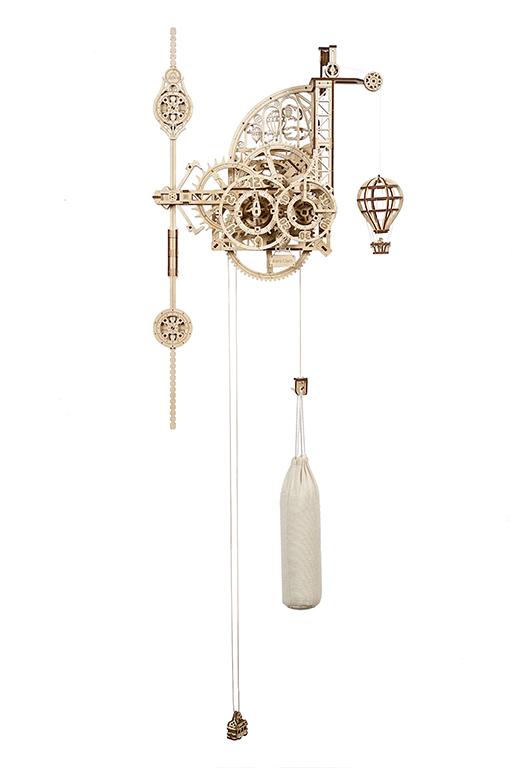This detailed color photograph features an intricate mechanical device that resembles a wall-hanging clock, crafted from gold-colored metal. Central to the device, a clock face is accompanied by a complex assembly of gears, numbering at least five. To the right of this gear arrangement, a delicate wheel suspends a small metal model of a hot air balloon. On the left, a vertical structure adorned with elaborately carved, weighted circles adds to the artistic complexity. Hanging below the middle cluster of gears is a gold-colored weight attached by a string. Additionally, another string to the right supports an oblong white pouch. The background of the image is white, highlighting the detailed craftsmanship of the device despite the slightly blurry, low-resolution quality of the photograph.